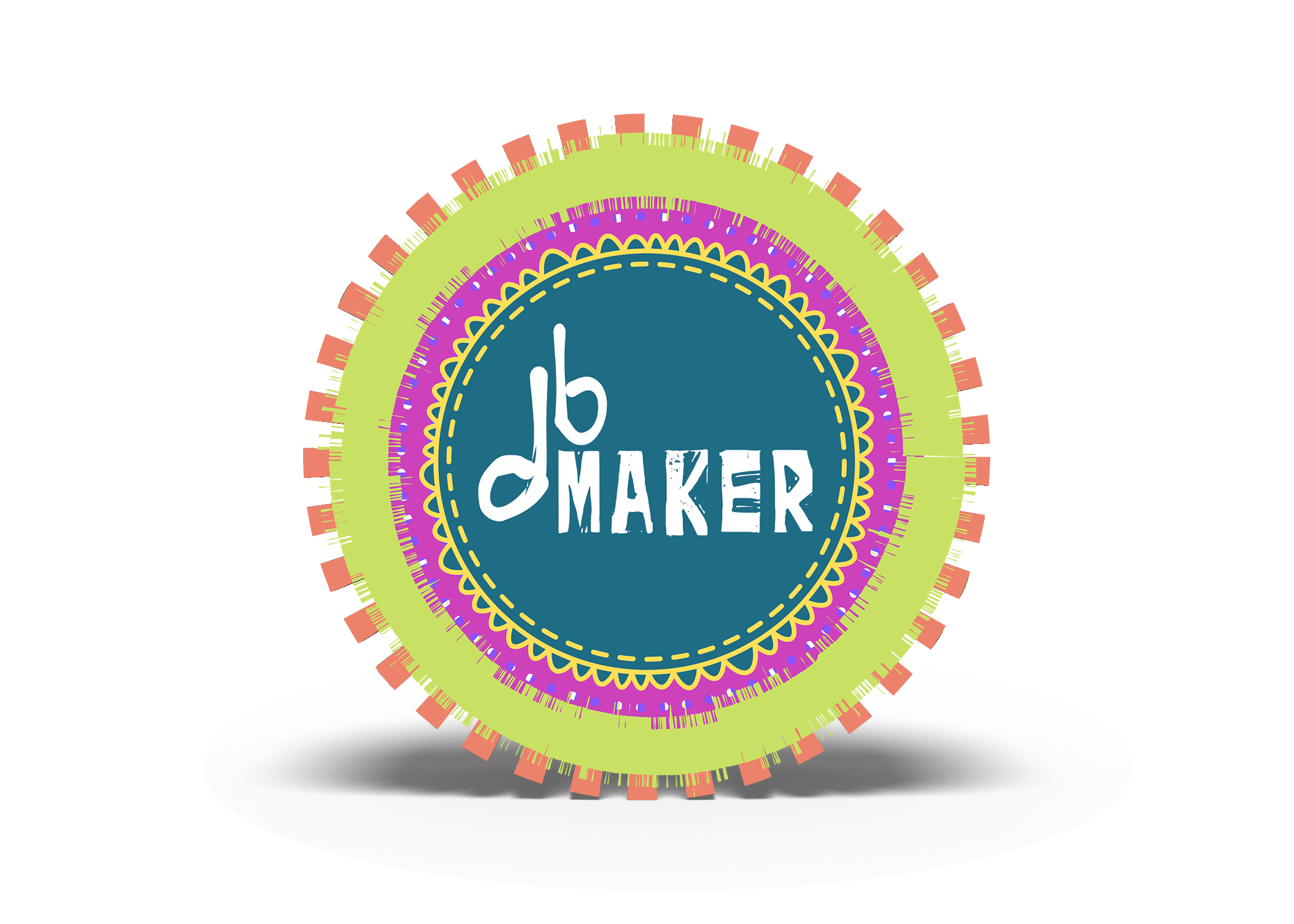The image features a large, prominent logo positioned centrally against a completely white background. The logo is circular, with intricate detailing and vibrant colors that fill the entire photo. The outermost part of the circle is adorned with evenly dispersed orange rectangles, reminiscent of cog teeth. Just inside this are concentric circles: a light green stripe, a light magenta stripe speckled with blue and white dots, and a medium blue circle outlined in yellow, which also features decorative yellow scrolls on its edges. Moving inward, there are yellow dashes punctuating the radius of another band. The very center is a dark green circle bordered by tiny, broken lines. Dominating the central space of this intricate design are the letters "D.B." resembling music notes, and the word "MAKER" in all capital white letters. The multi-colored palette includes shades of white, orange, green, purple, yellow, and blue. This intricate and colorful design suggests it is likely a corporate logo, potentially for a company named D.B. Maker, and could be the kind of logo seen on a business card.